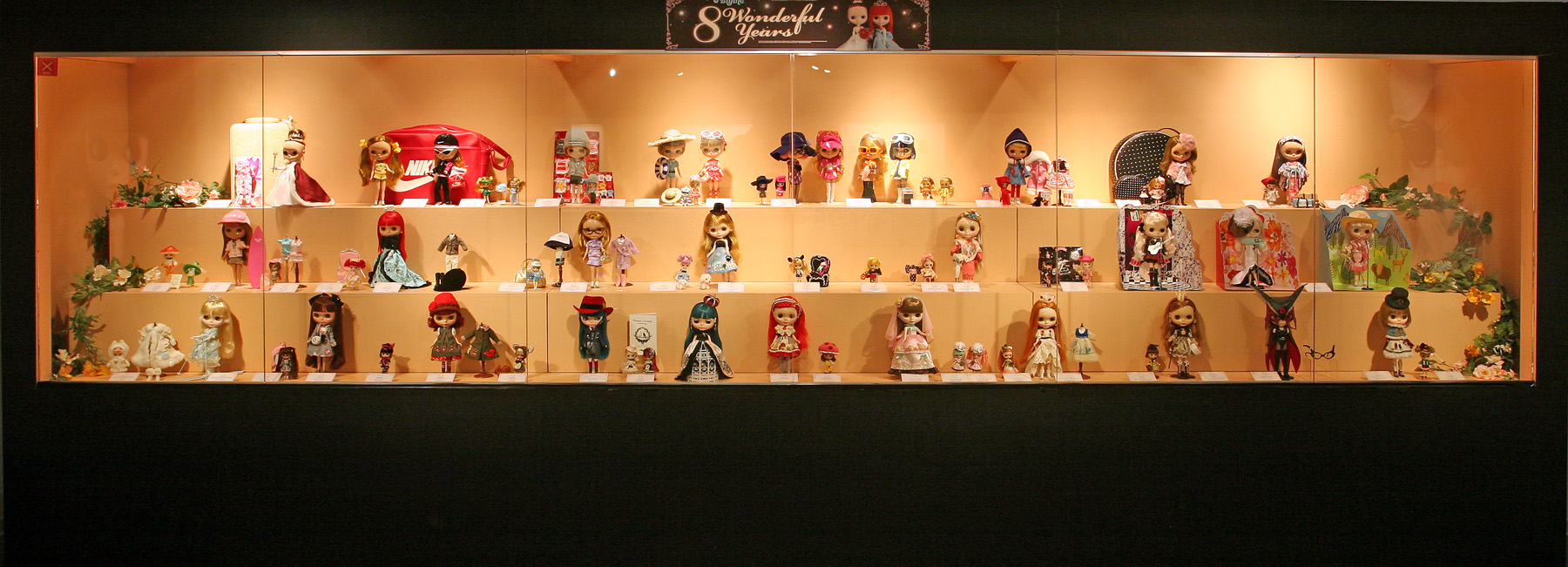This color photograph appears to be taken in a museum or store, showcasing a well-lit display case with a beige background. The rectangular glass case houses three shelves filled with dolls, most of which appear to be female, each adorned with various types of outfits and hair styles in different colors and lengths. The dolls, which resemble Madame Alexander or similar brands known for their large heads and small bodies, are accessorized and posed in different positions, primarily facing the observer. At the top center of the case, a black sign with gold lettering reads "Eight Wonderful Years," flanked by a picture of two dolls. Adding a touch of realism, there's an orange Nike bag visible towards the back left of the case. The display is illuminated by internal lighting, and some greenery decorates either end of the shelves, enhancing the overall presentation.